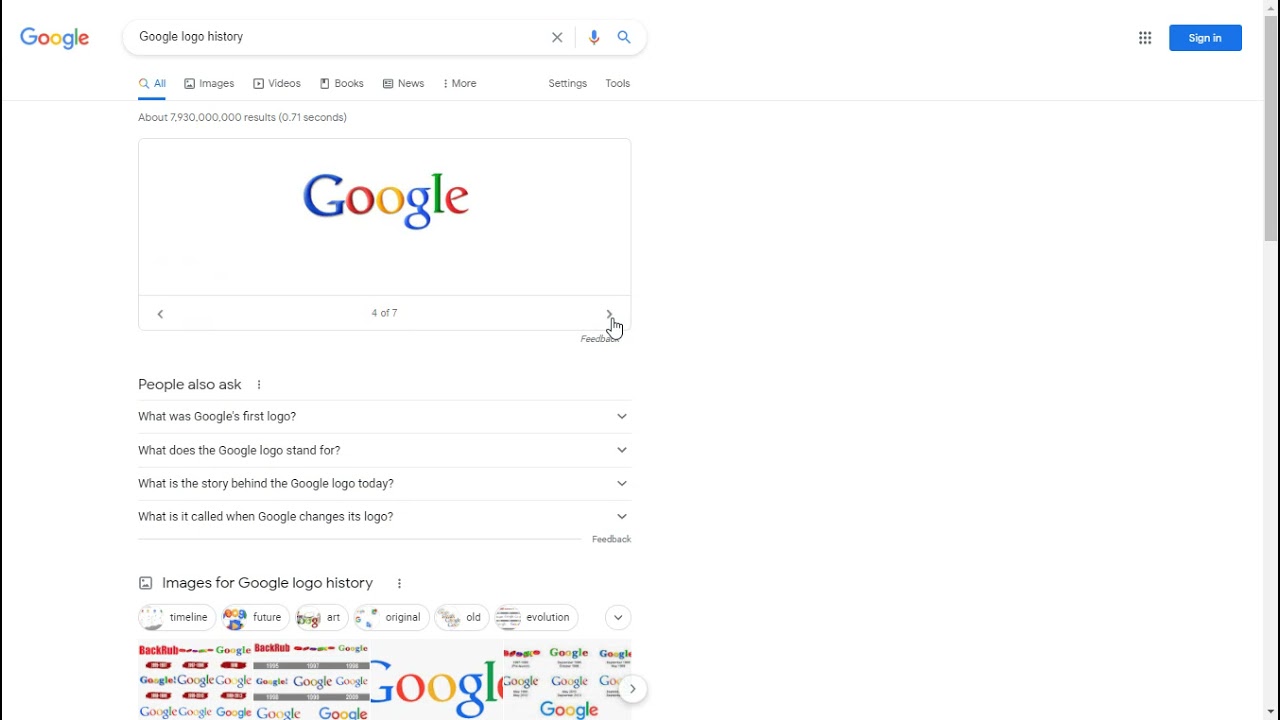This image is a detailed screenshot of a Google search results page displayed on a computer screen. At the top left, the recognizably colorful Google logo is prominently featured. To its right, the search bar contains the query "Google logo history" typed in black text. Adjacent to the search bar, there are several icons: an 'X' to clear the search, a microphone symbol for voice search, and the traditional magnifying glass icon for performing the search.

Beneath the search bar, a navigation menu allows users to filter their search results by categories such as All, Images, Videos, Books, News, and More. Additional navigation options include Settings and Tools. Just below this menu, a highlighted section displays the Google logo with a label indicating it is image four of seven in a carousel. Navigation arrows positioned to the left and right of this image enable users to scroll through the images.

Farther down the page, a "People also ask" section showcases a list of commonly asked questions related to the Google logo history. Below this section, a grid of various images depict the Google logo in different contexts and historical designs.